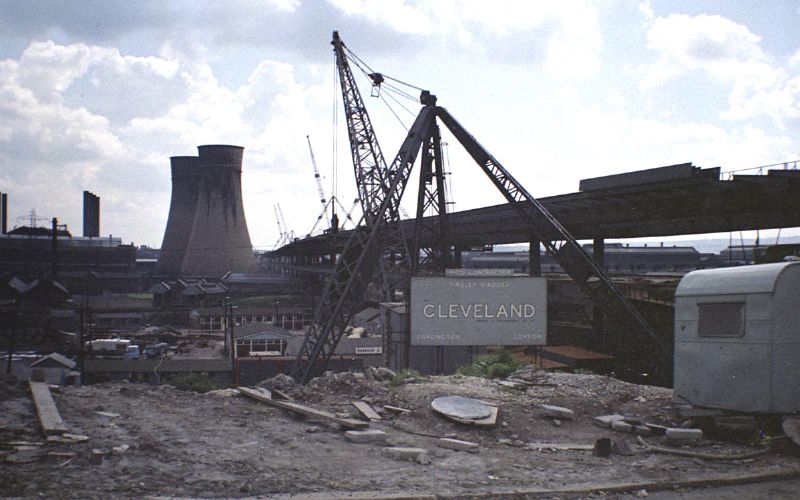The image displays an expansive, decrepit industrial site, possibly an old, abandoned nuclear or power plant. The foreground reveals a chaotic spread of construction debris, including beams and wood scattered across a gravel road that leads to what appears to be a deteriorating factory entrance. Prominently placed is a sign that reads "Cleveland," partially obscured by stone blocks and wooden planks. Flanking the sign are several tall cranes and low-lying, squat warehouses with large dock doors.

Towering over these buildings, a partially constructed bridge or walkway extends from the right towards the center of the image before disappearing, its structure seemingly abandoned mid-construction. Two prominent, large chimney-like structures, reminiscent of power plant smokestacks or water tanks, stand in the background, suggesting an industrial past. The sky occupies nearly half of the photo, displaying a serene blend of light blue and purple hues, dotted with fluffy white clouds, juxtaposing the gray, faded, and old-world tone of the site below. A camper trailer sits just at the edge of the frame, adding to the scene's sense of abandonment and desolation.